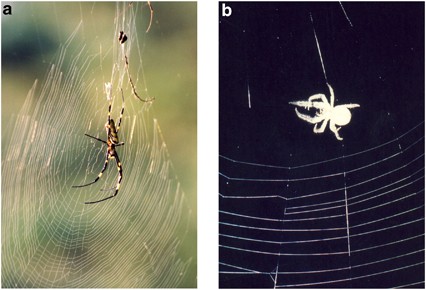The composite image features two vertically aligned, rectangular photos labeled 'a' and 'b' in lowercase letters in the upper left corners. The photo labeled 'a' on the left has a blurry green and brown outdoor background with a large, intricate spider web prominently displayed. The web consists of concentric circles and intersecting lines, creating small squares within its structure. At the center of the web hangs a spider with long legs. Its body appears brown and black, while its legs are yellow and black. There might also be a few bugs caught in the web. The image labeled 'b' on the right contrasts sharply with a solid black background and some horizontal white lines at the bottom, suggesting it was taken at night. The spider in this web has a stout, round body that is narrower at the top, appearing white overall, and it has noticeably shorter legs compared to the spider in the first image. This web also features vertical and horizontal lines, with the horizontal lines being slightly curved.